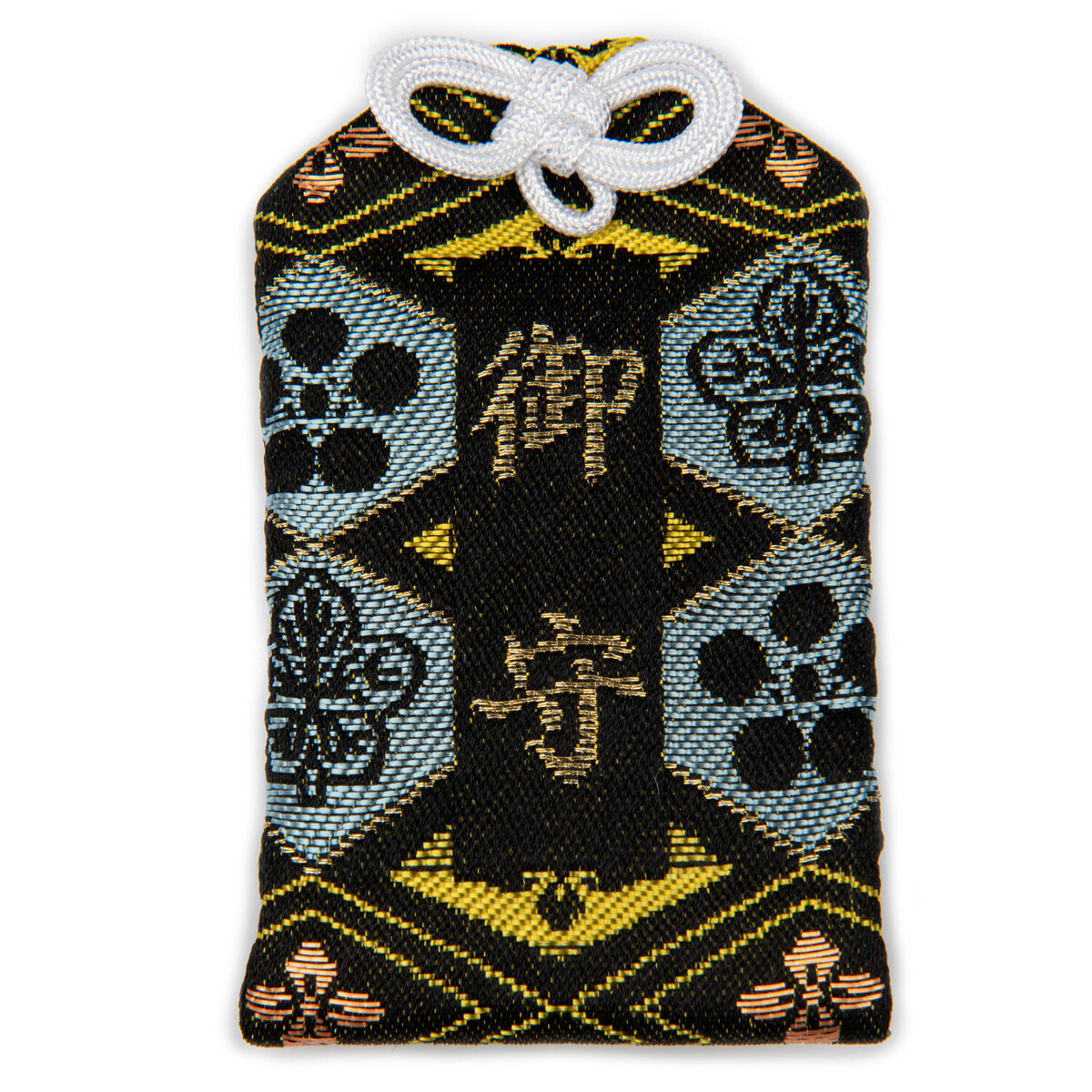The image depicts a small ornate fabric bag, likely used for holding keys or marbles. The bag features a woven white ribbon tie, resembling a decorative shoelace, at the top. In the center of the bag, a black vertical rectangle displays gold symbols, which may be Chinese or Mahjong characters. Surrounding the central area are intricate diamond-shaped patterns in blue, yellow, pink, and black, each containing designs reminiscent of paw prints, leaves, and flowers. The overall aesthetic combines vibrant colors and detailed motifs, giving the bag a unique and decorative appearance.